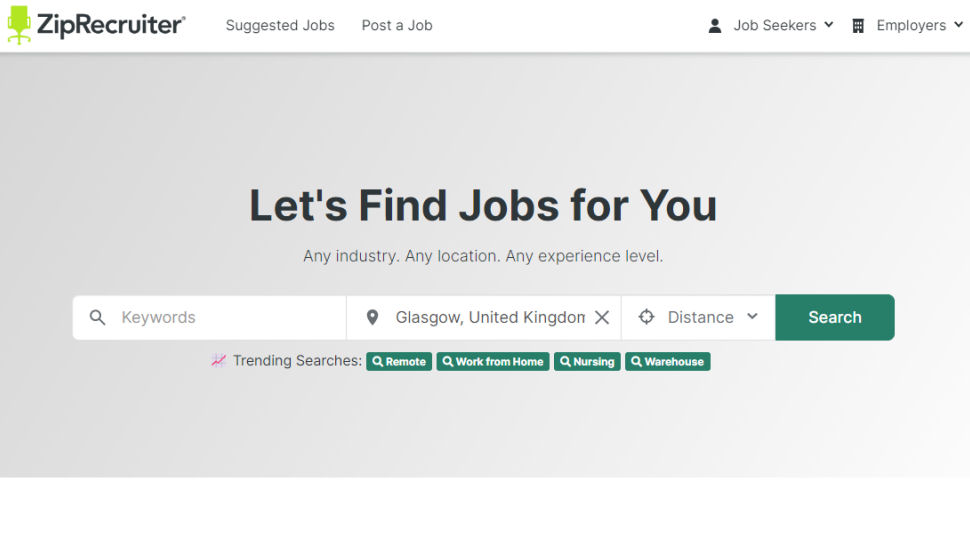This is a detailed screenshot of the ZipRecruiter website.

In the top left corner, the website prominently displays the company name "ZipRecruiter" alongside its logo, which depicts a bright neon green office chair facing forward. 

Adjacent to the logo and title, there are two primary navigation buttons: the first labeled "Suggested Jobs" and the second labeled "Post a Job." Following these options, there are two additional icons. The first is a small icon of a head and shoulders, labeled "Job Seekers," which includes a drop-down menu button for further navigation. Next to it is a small building icon labeled "Employers," also accompanied by a drop-down menu button. 

On a gray background beneath these navigation options, bold text reads, "Let's find jobs for you," followed by a subtext stating, "Any industry, any location, any experience level." Below this, there is a searchable text box for entering keywords, with a location field pre-filled with "Glasgow, United Kingdom." Adjacent to the location field, there is a drop-down menu button labeled "Distance," and a prominently placed "Search" button.

Further down the page, a list of trending job search terms is displayed, including popular queries such as "remote," "work from home," "nursing," and "warehouse."